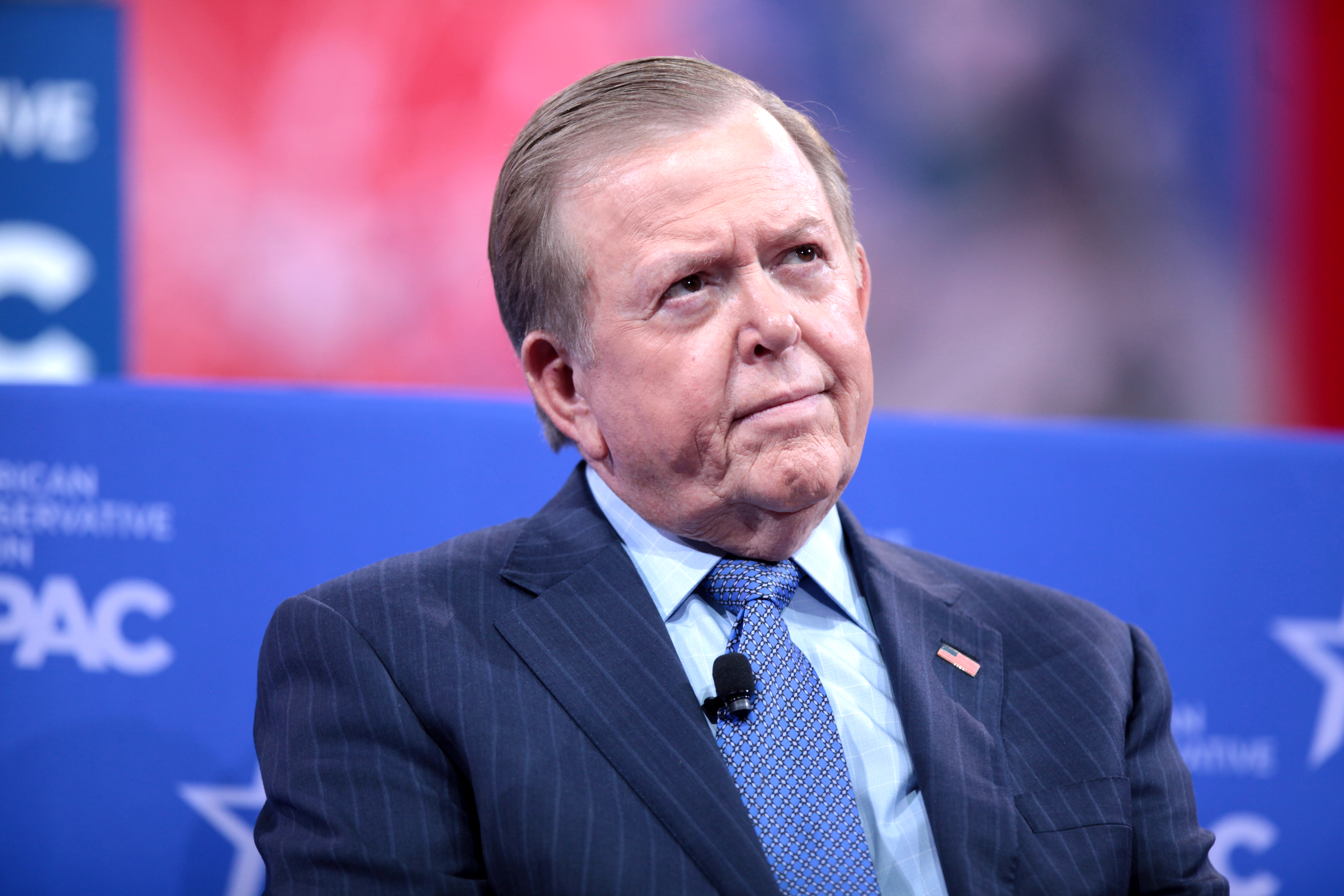The image is of an older, light-skinned man with medium brown hair, graying at the edges, and combed back. He has brown eyes and a slightly wrinkled face, giving off an appearance of attentiveness as he looks up and to the right, as if listening to someone speaking. He's dressed in a navy blue suit with a subtle pinstripe pattern, paired with a light blue shirt featuring a darker blue tie with a square pattern. On his left lapel, he proudly wears an American flag pin, and a black microphone is clipped to his tie. He is seated at the Conservative Political Action Conference (CPAC), identifiable by the blue background behind him adorned with white stars and the prominent "CPAC" sign. The background also features blurry elements with shades of red, white, and blue, indicative of the patriotic theme of the event.